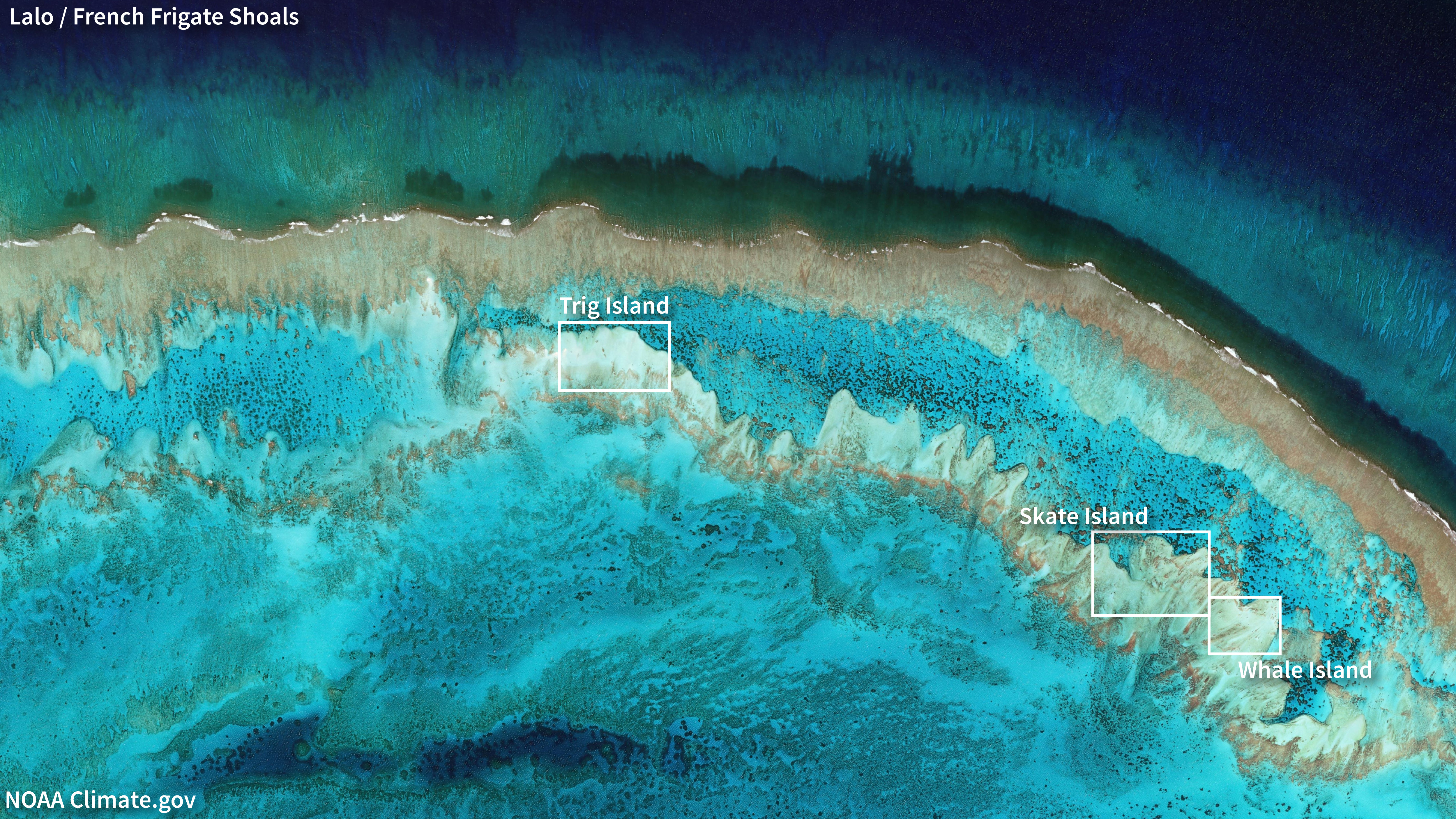The image presents a top-down, slightly blurry satellite view of the coastline of an island, labeled in the upper left corner as "Lalo, French Frigate Shoals," with "NOAAclimate.gov" marked in the lower left. This detailed composite features a series of interconnected landmasses, starting from a curved bluish strip of land a little below the upper left. This strip transitions into distinct, rocky, mountainous areas labeled as Trig Island in the center, and Skate Island and Whale Island towards the bottom right. The water surrounding these landforms exhibits a striking gradation of colors: deep blue at the top, transitioning to lighter blue, and finally a greenish-blue hue near the upper curve of the island. Each island is clearly demarcated with white boxes, providing a focused layout of the geographical features across this vivid, neon teal and light blue seascape.